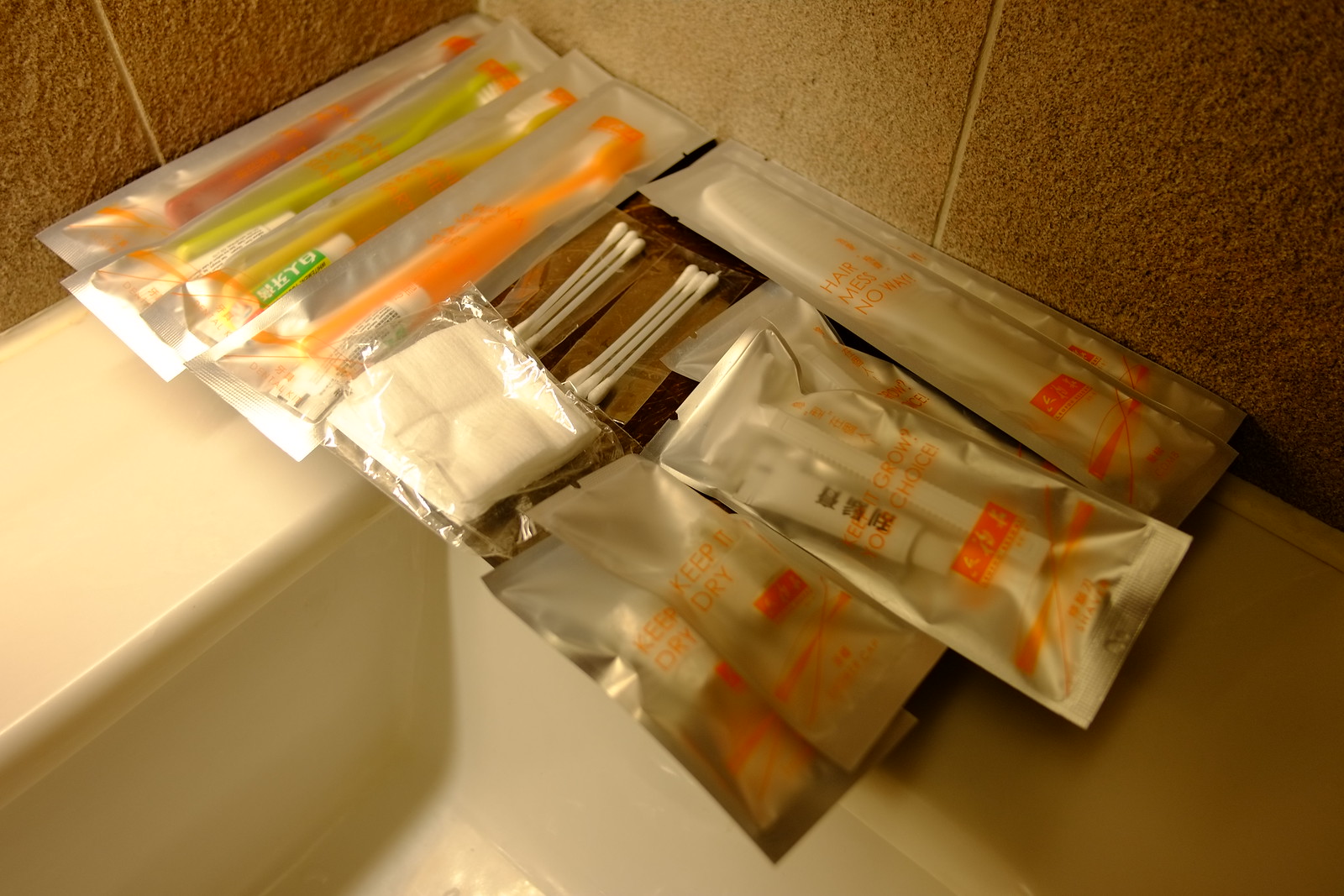This photograph showcases an assortment of neatly wrapped toiletries displayed on the ledge of a bathtub or sink, set against a backdrop of brown cement tiles. The ledge is white, providing a clean contrast to the packaging. Prominently featured are four individually wrapped toothbrushes with white bristles, distinguishable by their different colored handles—orange, green, yellow, and a lighter shade of orange. Each toothbrush is enclosed in a bag that's silver on one side and clear on the other, allowing visibility of green Japanese characters and additional orange writing. Accompanying these are a set of toiletries including a clear bag with a white comb labeled "hair, mess, no" in orange font, a small white razor, and a tube of shaving cream marked with the slogan "keep growing? Your choice." A bag of tissues, a pack of four white Q-tips, and a couple of indistinct packages are also present, with one of the ambiguous packages bearing the label "keep dry," potentially housing a shower cap. The entire arrangement gives off the impression of items provided to guests at a hotel, meticulously organized and aesthetically presented.